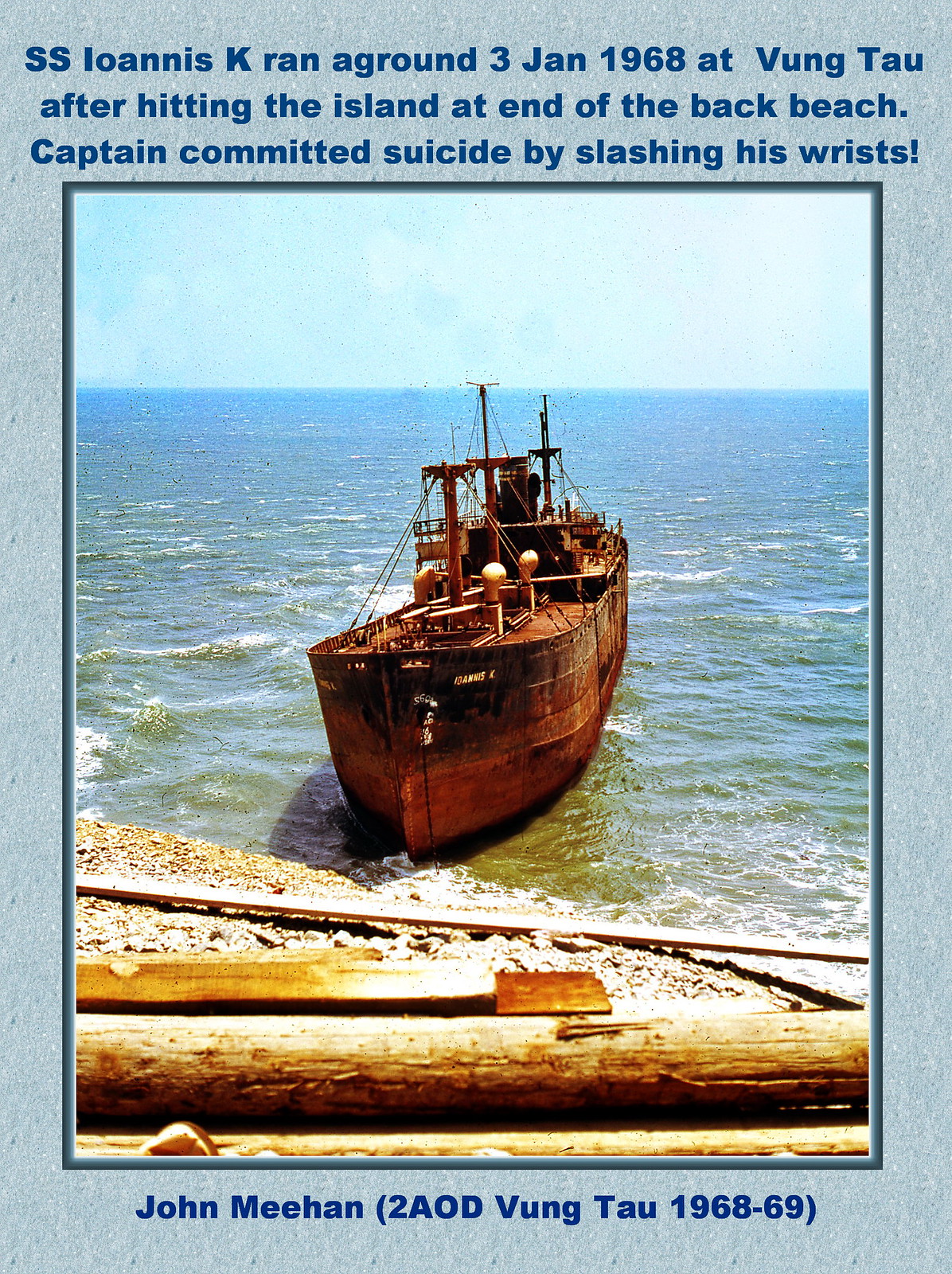The image depicts an aged wooden shipping vessel, resembling an ark, partially run aground near a sandy, rocky shore with scattered wood planks and tree logs. The boat, seemingly in great disrepair with brown, discolored wood, is lodged in shallow, light-turquoise water of a large sea with no land visible on the horizon. The vessel, identified as SS Ionis K., ran aground on January 3, 1968, at Vung Tau after hitting an island at the end of the back beach. Tragically, the captain committed suicide by slashing his wrists. The borders of the photograph contain explanatory text: above the image, it reads "SS Ionis K ran aground 3 Jan 1968 at Vung Tau after hitting the island at end of the back beach. Captain committed suicide by slashing his wrists." At the bottom, "John Meehan, 2AOD Vung Tau 1968-69" is inscribed.